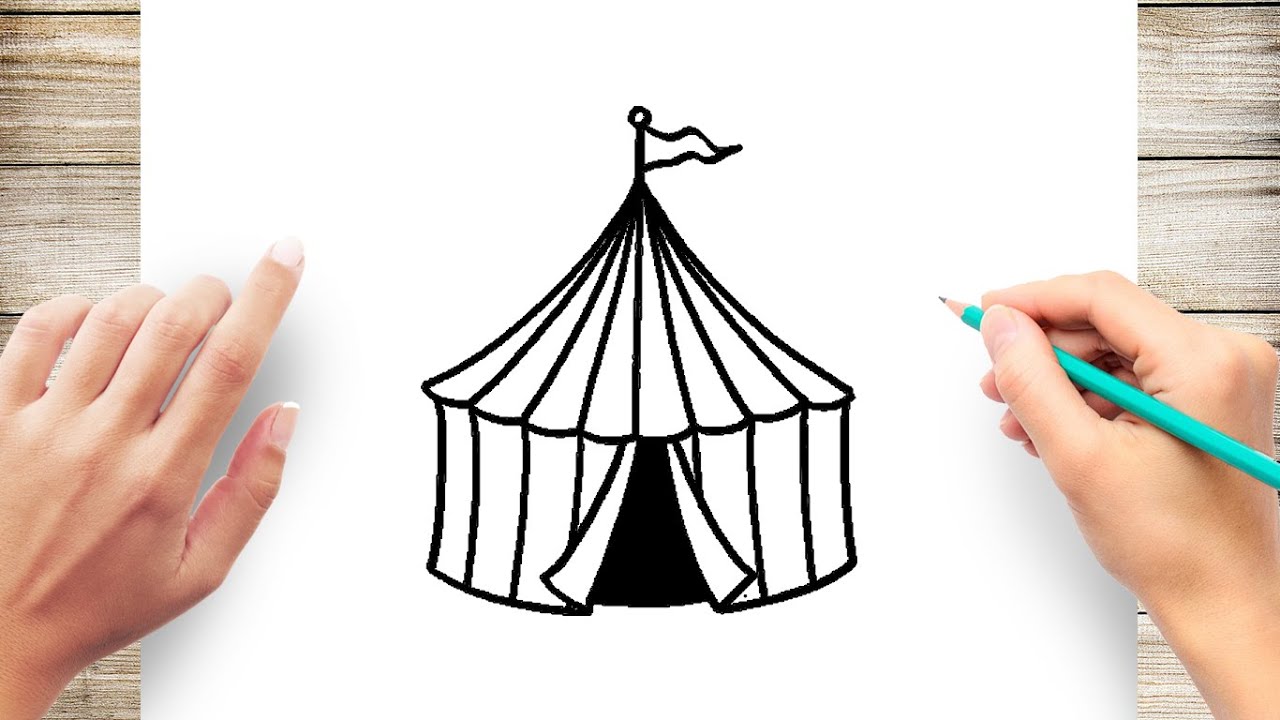This detailed color photograph captures a flat-lay scene where two Caucasian hands are actively engaged in drawing a black and white circus tent on a piece of white paper. The background showcases a horizontal layout of brown wooden planks. In the center of the image is the piece of white paper, with the left hand positioned to hold it in place, and the right hand wielding a teal-colored pencil. 

The tent illustration, done in black lines, is prominently featured in the middle of the paper. The tent itself is cylindrical with a triangular, peaked rooftop, segmented into variegated black and white sections. At the apex of the roof, a thin flagpole extends upwards, topped by a small ball and fluttering a pennant-style flag to the right. The front of the tent is designed with open flaps, revealing a dark interior. The overall photograph highlights the meticulous detail and artistic process, showcasing the hands-on creation of this intricate circus tent drawing.